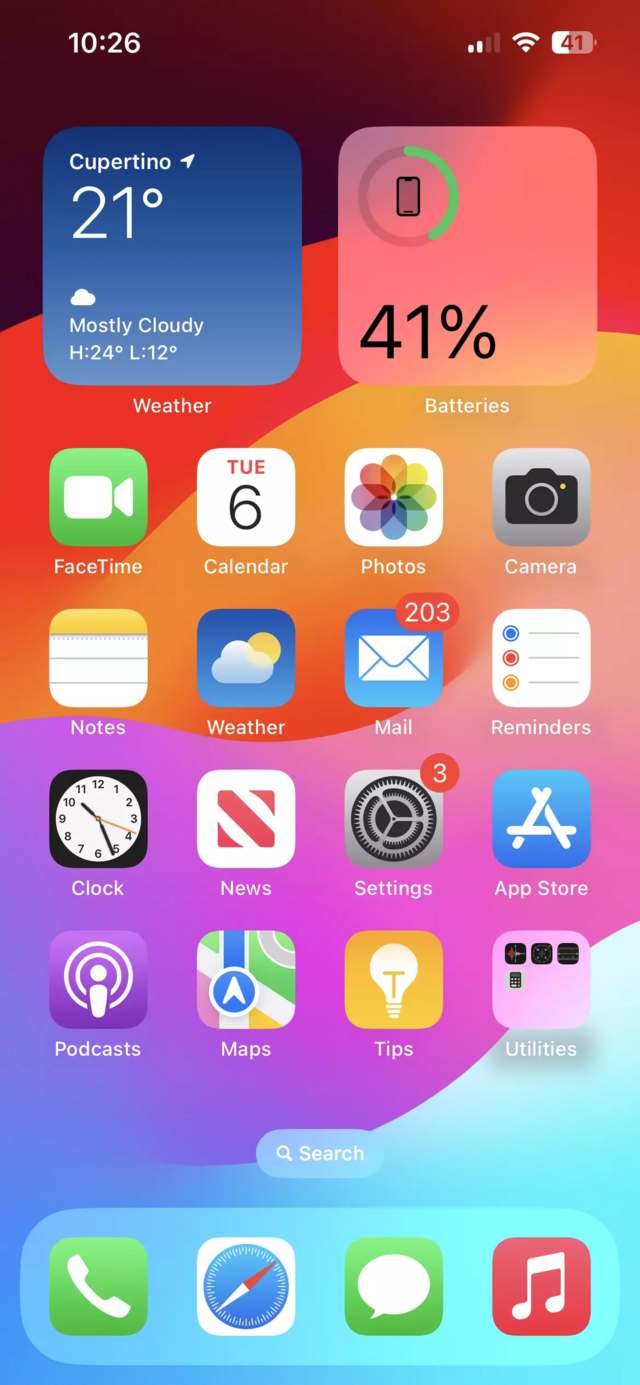The image portrays an iPhone screen with a vibrant gradient background. The color scheme begins with a near-black at the top left, shifting diagonally into rich red, then transitioning into a vivid orange reminiscent of a sunset. This orangish hue smoothly melds into a deep purple before finally blending into a stunning gradient of blue that lightens as it descends.

At the top of the screen, the current time is displayed in white font as "10:26," flanked by two bars of cellular service and a full Wi-Fi signal on the right. Additionally, the battery icon, also white, indicates a 41% charge remaining.

Below this, the first widget is a blue gradient box featuring white text. It shows the weather information: "Cupertino," a temperature of "21°C," and a small cloud icon accompanied by the text "Mostly cloudy, H 24°C, L 12°C." Adjacent to this widget is a semi-transparent widget displaying a 41% battery charge in black font along with a visual representation of the remaining battery life.